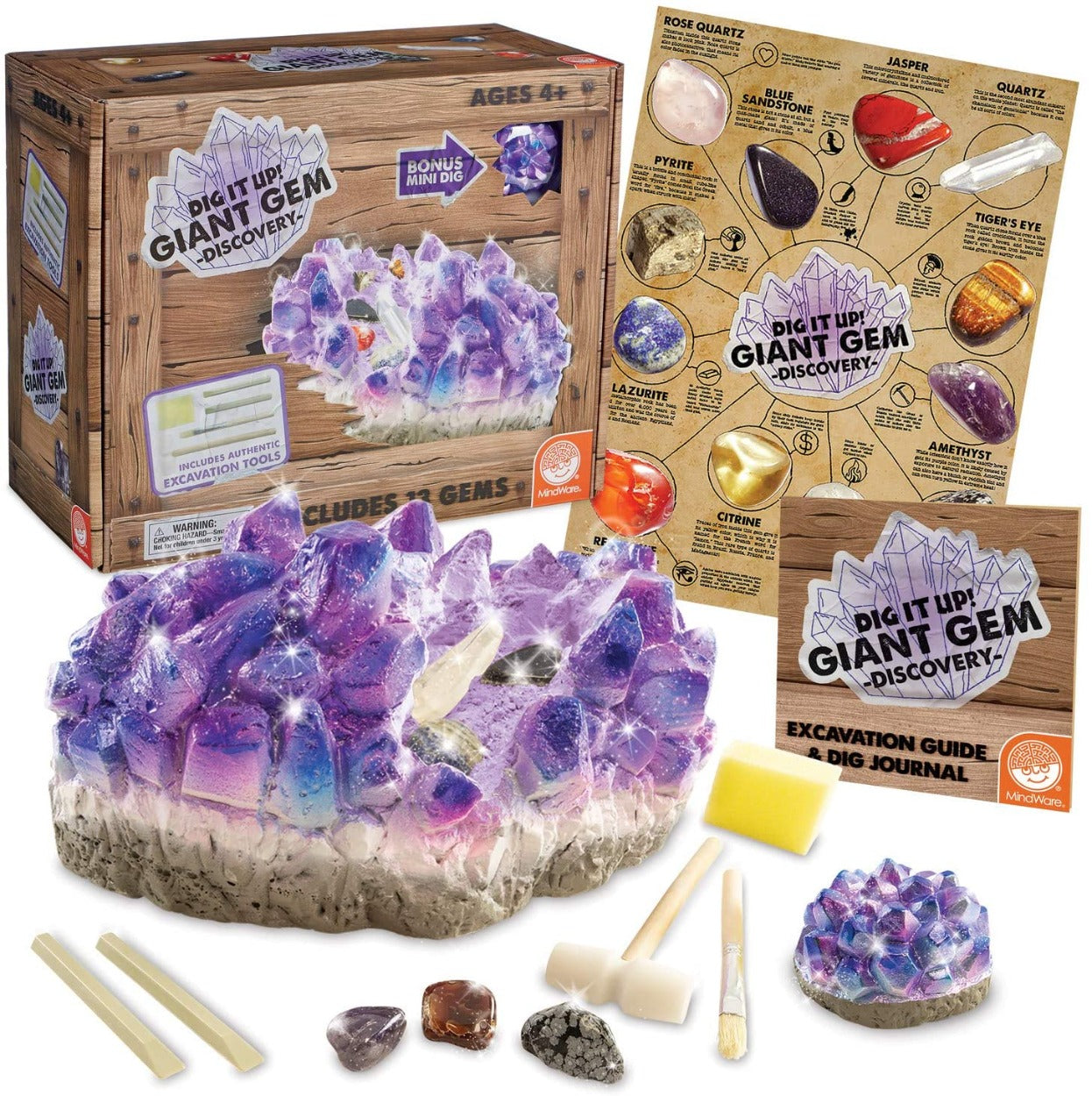This image is an advertisement for the "Dig It Up Giant Gem Discovery" kit, designed for children aged 4 and up. The background features a cardboard box styled like a wooden crate, adorned with a logo of purple crystals and text that highlights a "Bonus Mini Dig." Adjacent to the box is a detailed chart that lists potential discoveries, including Rose Quartz, Blue Sandstone, Jasper, Quartz, Tiger's Eye, Amethyst, Citrine, Lazurite, and Pyrite. The foreground displays a large, purplish crystal resembling part of a geode, surrounded by excavation tools such as a mallet, chisels, a brush, and a yellow sponge. The kit seems to include authentic excavation tools and a booklet titled "Dig It Up Giant Gem Discovery Excavation Guide and Dig Journal."